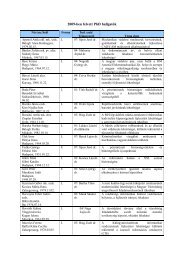The image depicts a low-resolution, pixelated chart or table that appears to be from an Excel or PDF document. Despite zooming in, the text remains indecipherable due to the poor quality of the image. The chart consists of four columns and approximately 17 to 18 rows, each separated by bold black lines. The topmost row, which serves as the header, is highlighted in blue, and there is a black text header above this blue section that is also unreadable. The image background is white, and while the chart has black borders, the only other color present is in the blue header row. Notably, every entry in the second column contains the number one. The overall structure resembles an ingredients list or a nutrition label, but the exact contents are unclear.